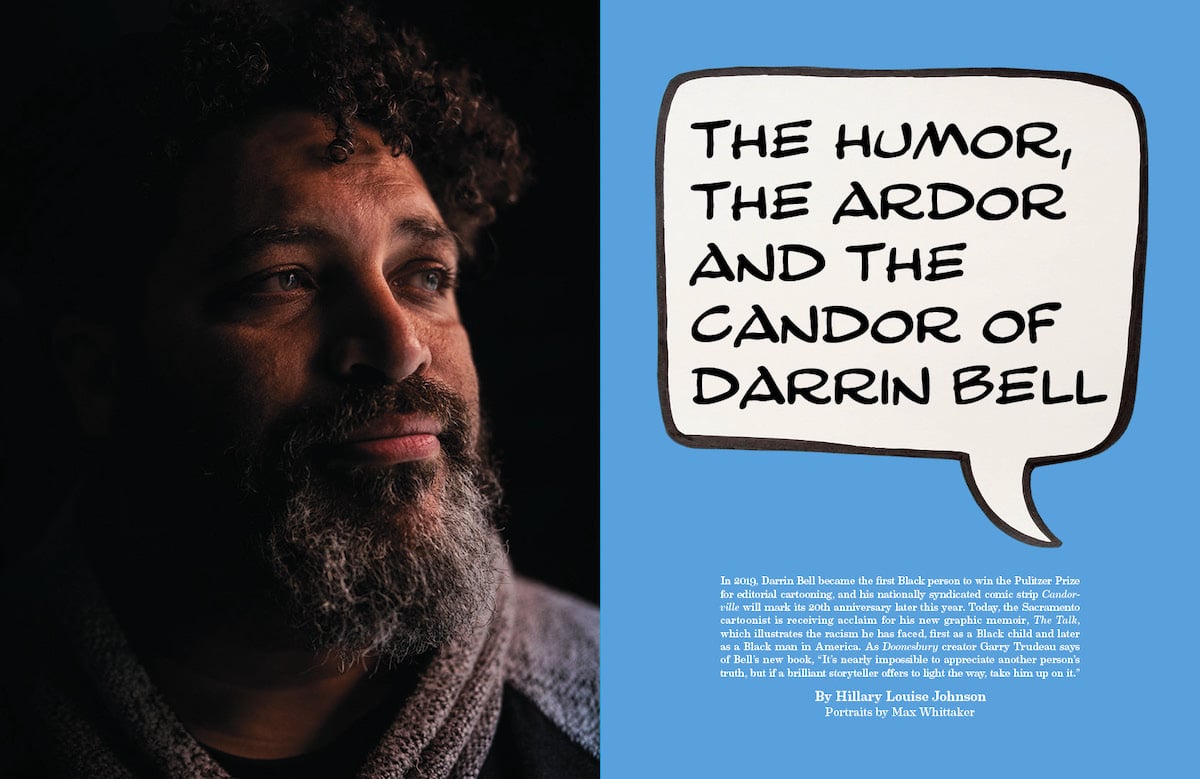The image is a graphic featuring a photograph of a man with light brown skin, curly medium-length dark hair, and a semi-white beard. He is slightly smiling and looking off to the right, with his face illuminated from that direction. He appears to be wearing a gray scarf, and the left side behind him fades into darkness. On the right half of the graphic, there is a blue background with a white speech bubble outlined in black. Inside the speech bubble, in comic strip style text, it says, "The humor, the ardor, the candor of Darren Bell." Beneath this in very small text, it reads: "In 2019, Darren Bell became the first Black person to win the Pulitzer Prize for editorial cartooning, and his nationally syndicated comic strip, Conjure, will mark its 20th anniversary later this year. Today, the Sacramento cartoonist is receiving acclaim for his new graphic memoir, The Talk, which illustrates the racism he has faced—first as a Black child and later as a Black man in America." A quote from Doonesbury creator Gary Trudeau follows: "It's nearly impossible to appreciate another person's truth, but if a brilliant storyteller offers to light the way, take him up on it." The text concludes with "By Hilary Louise Johnson, portraits by Max Whitaker."